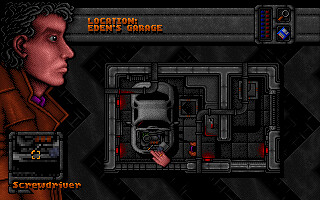The image presents a detailed scene from a video game design. Dominating the left side is a character portrayed from the torso up, wearing a brown trench coat. The character's face is seen in profile, featuring curly gray hair and a purplish-pink complexion. Adjacent to the character's face is a gray square displaying an orange picture icon with the text "Screwdriver" below it in orange.

To the right of the character, a platform is visible. Above this platform, "Location: Eden's Garage" is inscribed in orange text, separated by a gray horizontal barrier. The scene also includes various gadgets, such as blue and red bullets, a magnifying glass, and a blue square.

Beneath the platform, part of a gray vehicle is visible, its structure marked by pipes and edged with red lights. The overall background of the image is a blend of black and gray tones.